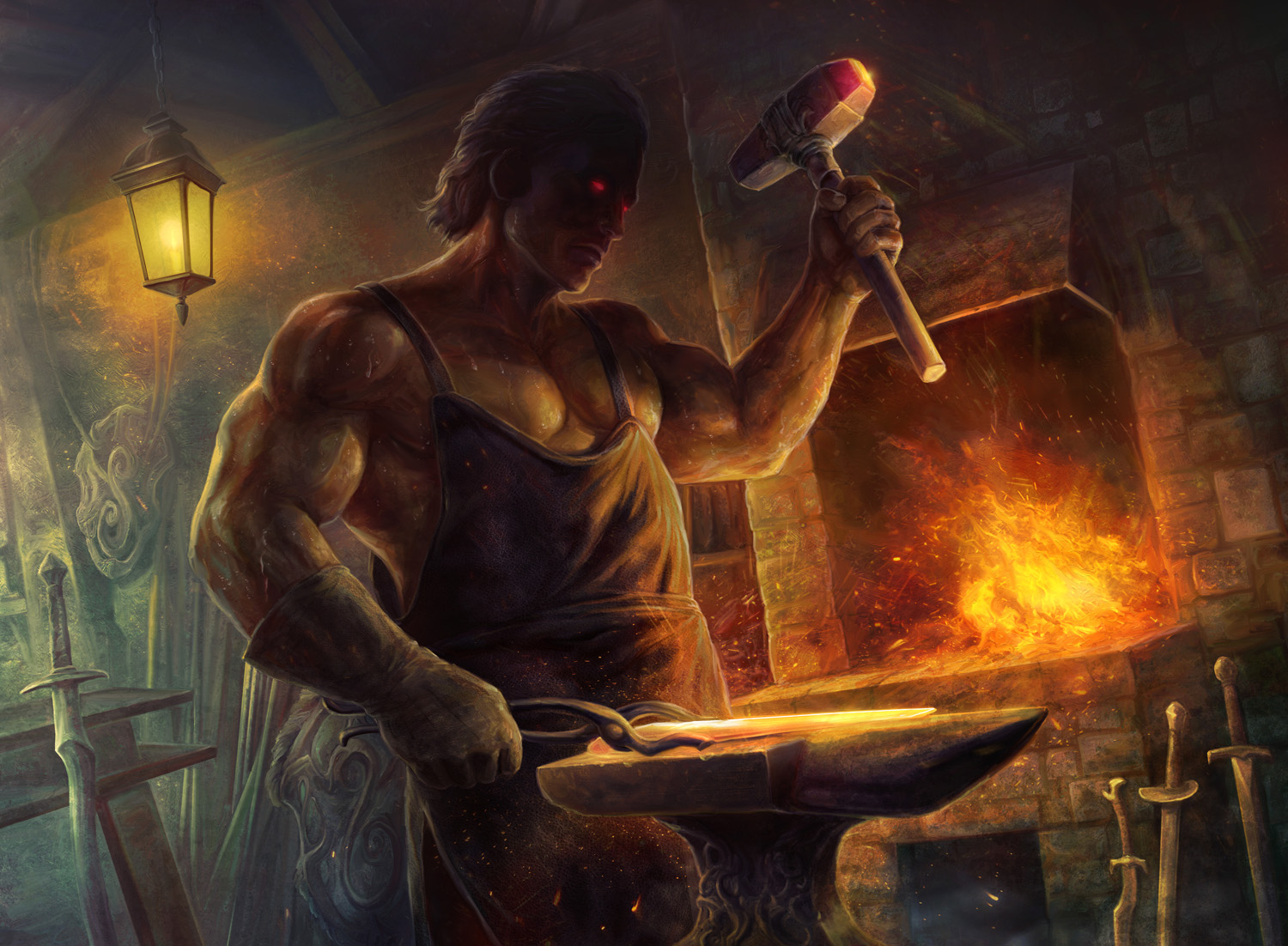The image depicts a brawny blacksmith from an ancient era, captured possibly as a piece of artwork or a snippet from a gaming web page. The scene is vibrant and detailed, with a robust, shirtless man standing at the center, showcasing his well-defined muscles. He wears a heavy apron that complements his hardened physique and black gloves that extend almost to his elbows. The blacksmith's left hand is raised, holding a gavel-like hammer with a heated, orangish-yellow metal end, while his right hand grips a pair of tongs clamped onto a glowing, metallic piece. His eyes have a mesmerizing orange glow. Behind him, a lit stone fireplace casts a warm, fiery light, enhancing the overall intensity of the image. Additional details include a sword leaning against a table, various blacksmithing tools scattered around, a fire stoked near the right, and a lantern light illuminating the scene.